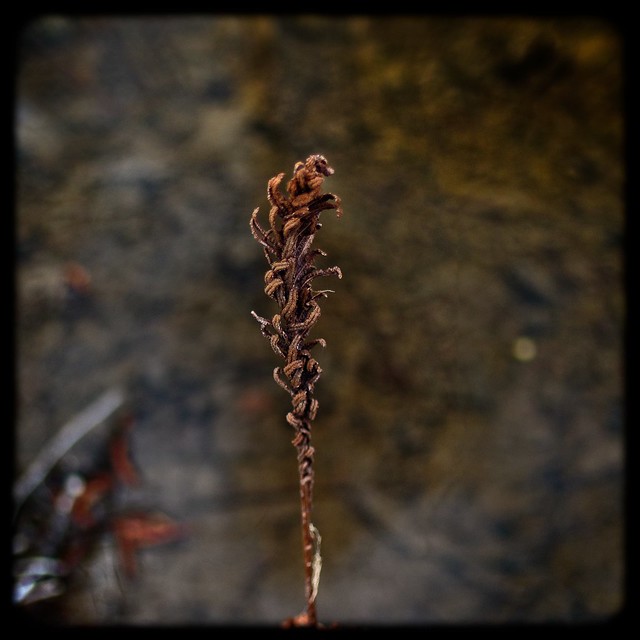The photograph captures a detailed, close-up view of a tall, thin plant, likely a type of reed or dried vegetation, prominently set against a blurry, indistinct background. The main subject of the image is a brown-colored plant with a slender stem that emerges from the soil and extends vertically. As the stem rises, it is initially bare, but further up it becomes adorned with a number of small, curled leaves or fronds, which vary in shade from light brown to dark brown. These leaves create a clustered, almost bud-like appearance towards the top. The background, bathed in brown tones with patches of gray and hints of out-of-focus black, red, and silver objects, gradually fades to black around the edges, further drawing attention to the plant. This daylight shot, likely taken on an overcast day due to the diffuse lighting and muted colors, highlights the intricate textures and forms of the plant's dried leaves, offering a stark yet evocative glimpse of nature's subtle details.